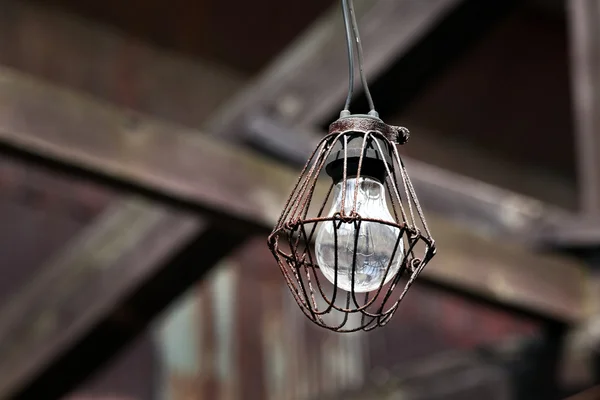The image captures a detailed close-up of a vintage light bulb hanging upside down by a black cable. The light bulb is encased in a rusted wire cage, giving it a distinctly weathered and industrial look. The surrounding environment, although out of focus, suggests an old barn or tin shed warehouse, characterized by wooden slats and possibly rusted corrugated metal in the background. The backdrop, hued in lighter brown tones with visible gray and brown ceiling beams, provides a textured contrast to the sharply focused centerpiece. The entire scene evokes a rustic, postmodern aesthetic, blending elements of decay and industrial design.